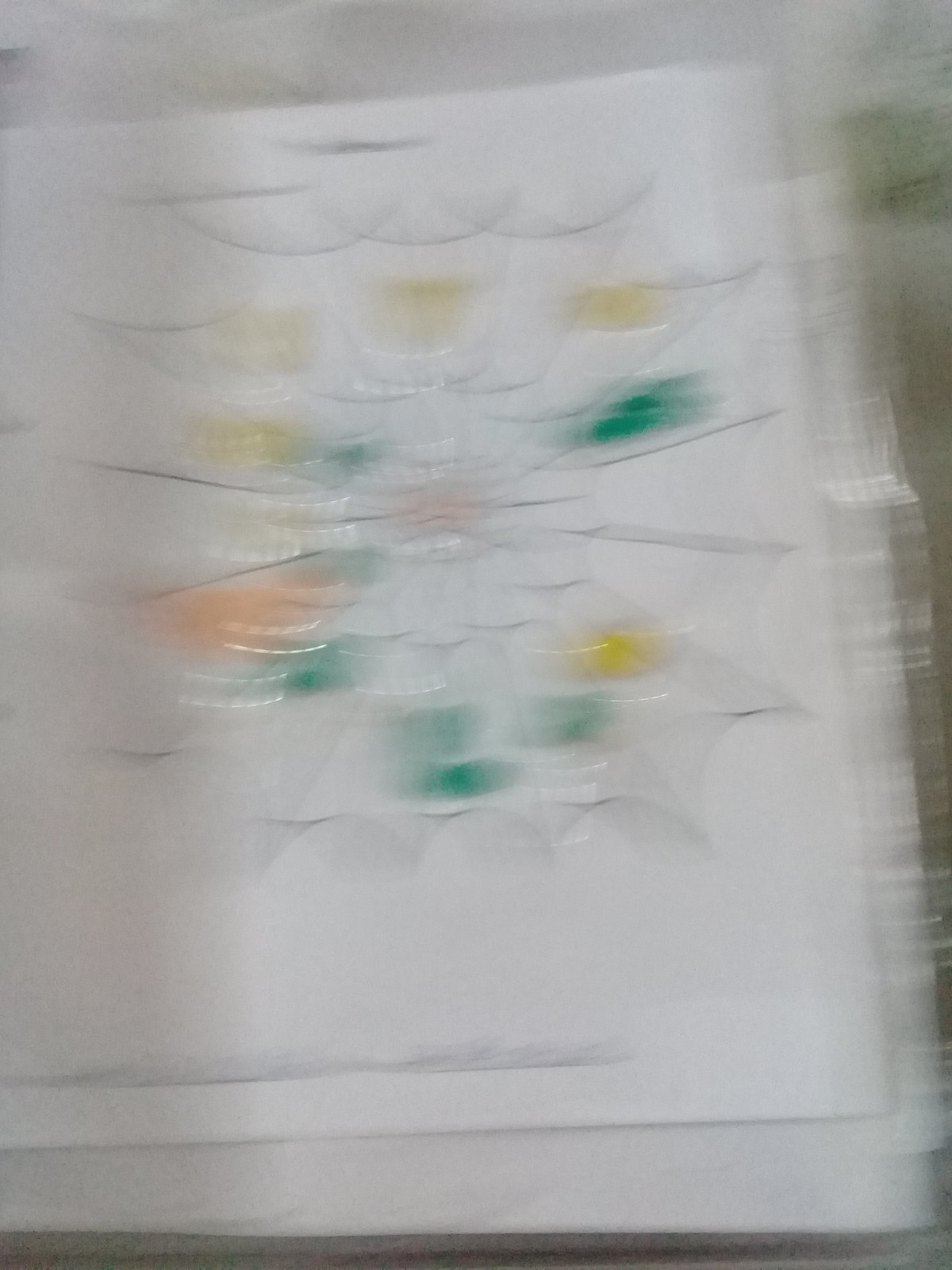The image depicts an extremely blurry photo of what appears to be a child's coloring worksheet on a blank white piece of paper. Despite the poor quality and motion blur, the central focus seems to be a drawing resembling either a spider web or a flower, composed mostly of gray lines that suggest pencil work. Scattered across the drawing are various blobs of color, including six or seven green smudges, five yellow spots, and one or two orange marks, which might be attempts at coloring by the child. There is a faint red circle in the middle of the drawing, adding to the ambiguity of whether it represents a web or a flower. At the bottom of the page, partially readable writing likely includes the child's name, combining printed and handwritten text. The edges of the photo have darker areas, indicating that the paper might be laying on a table or the floor. The top of the page also contains some blurred, unreadable text, further contributing to the overall vagueness of the image.